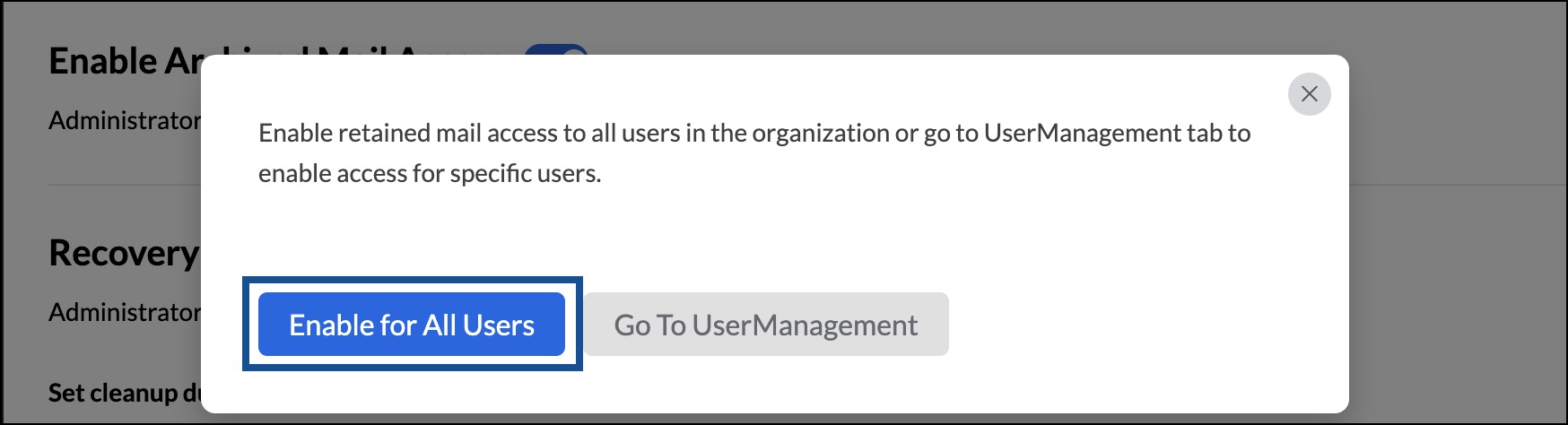In the image, a prominent pop-up text box predominantly covers the background, rendering it nearly invisible. The pop-up has a clean white background with black text. Faintly visible behind the pop-up are the words "Enable Administrator," "Recovery Administrator," and "Start Setup Cleanup Disk," hinting at a broader administrative interface.

The black text on the pop-up reads: "Enable retained mail access to all users in the organization or go to the User Management tab to enable access for specific users." Below this instruction, two clickable options are presented. On the left, a blue button with white text displays "Enable All Users," which is the currently selected option, as indicated by a blue square around it. On the right, a gray button with black text reads "Go to User Management," which remains unselected.

Additionally, a small, black 'X' within a gray circle is positioned in the top-right corner of the pop-up box, serving as the close icon for the pop-up interface.